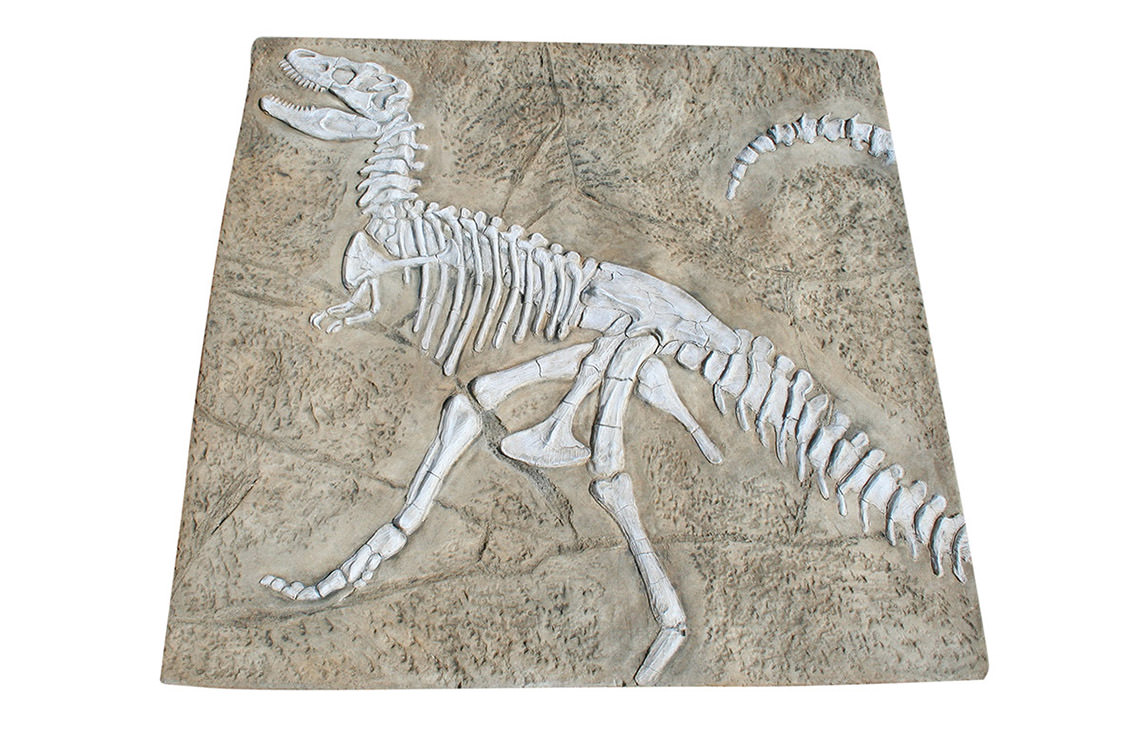The image portrays a highly detailed and intact dinosaur fossil, embedded in a rock-like material that is predominantly tan and gray in color. The fossil itself is stark white, contrasting sharply with its surrounding. The dinosaur, which could be a raptor or a t-rex, is depicted standing on its two hind legs with its head in the upper left corner, mouth open to expose a set of sharp, elongated teeth. Its small front arms are raised, indicative of its standing posture. The creature's long tail exhibits a distinctive curve, extending downward and then swooping up, with the tip visible in the upper right corner of the image. Engraved lines or patterns intersect the rock surface, adding texture and depth to the scene. The fossil is remarkably well-preserved, showcasing intricate details such as rib bones, vertebrae, pelvic bones, and even its front claws. The lifelike pose and meticulous preservation offer a vivid glimpse into the ancient past.